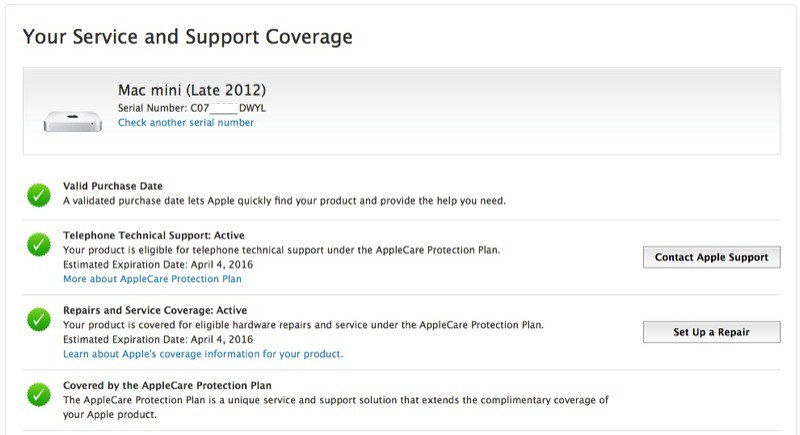The image is a screenshot of an Apple support and service coverage page for a Mac Mini (late 2012) device. The screenshot features a horizontally aligned, rectangular interface with a light gray border. At the upper left-hand corner, the header reads "Your service and support coverage" accompanied by an image of a Mac Mini displaying the Apple logo. Below this, the text specifies "Mac Mini (late 2012)" along with a serial number and a blue link labeled "Check another serial number."

On the left side of the screenshot, there are four green circles with white check marks arranged vertically. The first check mark is labeled "Valid purchase date," explaining that this helps Apple quickly identify the product and provide assistance. The second check mark indicates "Telephone technical support active," noting that the product is eligible for telephone technical support under the Apple Care Protection Plan, with an estimated expiration date of April 4, 2016. Adjacent to this, there is a blue link, "More about Apple Care Protection Plan," and a button labeled "Contact Apple support."

The third check mark states "Repairs and service coverage active," confirming that the device is covered for eligible hardware repairs and service under the Apple Care Protection Plan, with the same expiration date of April 4, 2016. A blue link next to this reads "Learn about Apple's coverage information for your product" and is accompanied by a button "Set up a repair."

The final check mark at the bottom reiterates that the product is "Covered by the Apple Care Protection Plan," highlighting that this plan extends the complimentary coverage of the Apple product. The overall color scheme for the interface is primarily white, black, gray, blue, and green. The majority of the text content appears aligned on the left side, occupying most of the screenshot, and emphasizes the service and support details for the Mac Mini.